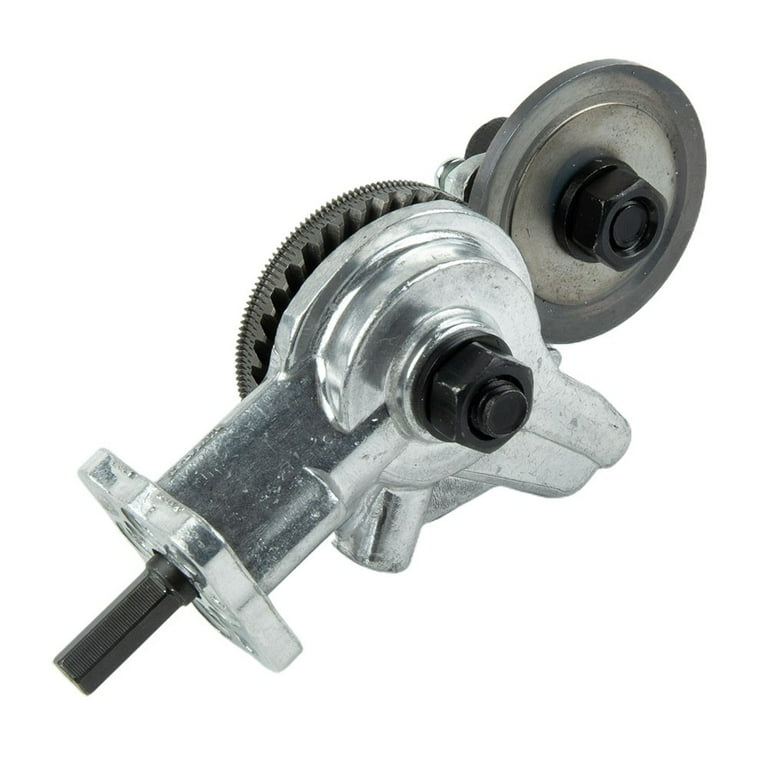The image depicts a detailed, intricate mechanical device primarily composed of metal components. In the upper right corner, there's a cylindrical black wheel featuring a black screw nut at its center, which appears to be connected to a flywheel. This flywheel is linked to a silver cylindrical area, the lower end of which extends outwards to a tapered black nozzle. This nozzle protrudes from a silver square piece and is oriented towards the bottom left corner of the image. Along the cylinder, there are multiple black screws. Additionally, on the left side of the cylindrical structure, there seems to be an axle or gear mechanism with visible gray teeth, possibly allowing rotational movement. The entire assembly, against a white background, showcases an intricate interplay of black and silver metallic parts interlocked with bolts and screws, suggesting its role in some precise mechanical function.